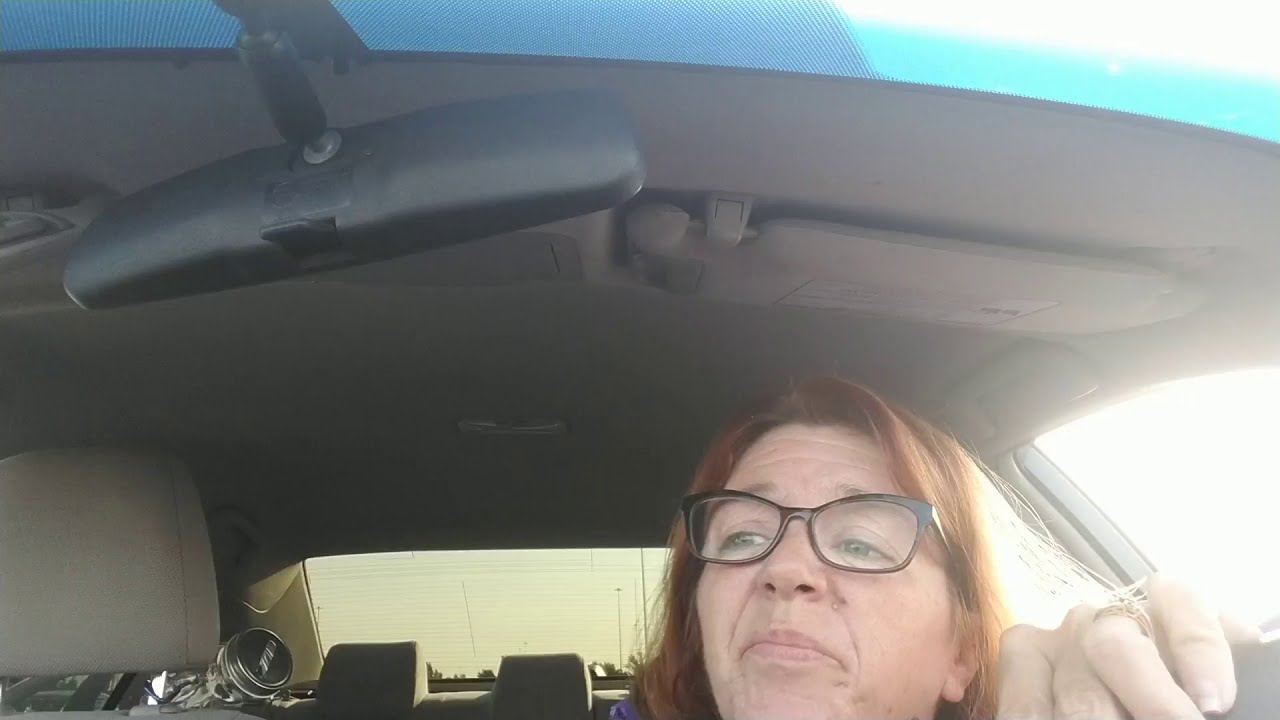In the image captured from dash cam footage, you see a woman in her 50s or early 60s with chin-length, reddish-brown hair, situated inside a car during daylight. The dash cam is positioned improperly, focused too high, resulting in the car’s gray interior roof being prominently displayed. The woman, located toward the bottom right of the frame, is wearing black, circular glasses with slightly thick frames, and her green eyes are directed to her front and right, possibly at the dashboard. She maintains a straight, neutral expression. Her left hand, adorned with a wedding ring on her ring finger, rests on the steering wheel. The image also shows the car's front passenger seat headrest, the rearview mirror in the upper left, and the back window with headrests visible in front of it. Various items, including something silvery, are placed behind the passenger seat. The sun can be seen shining brightly in the car, casting light over her left shoulder. The interior colors of the car include shades of brown, blue, yellow, black, green, and purple.